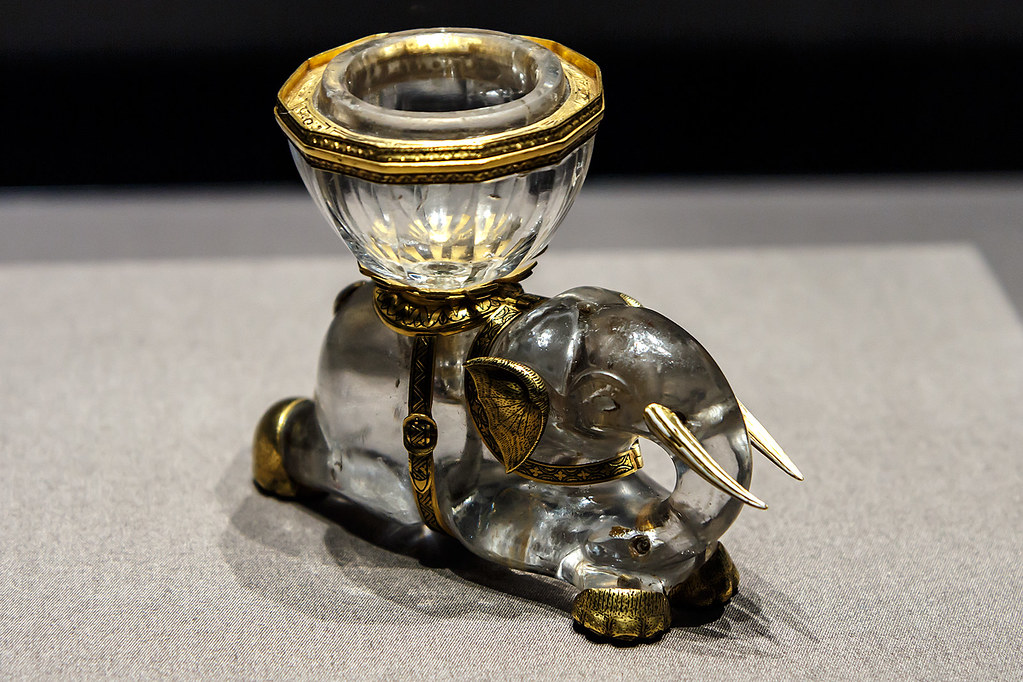This photograph showcases a delicate elephant figurine crafted from translucent glass. The figurine is adorned with intricate gold embellishments, including gold tusks, ears, and feet, and rests on a gold platform. Positioned in a reclining pose, the elephant is also outfitted with a beautifully detailed gold saddle that wraps around its body. Atop the saddle sits a relatively large glass bowl, sized at approximately one to two inches in diameter, with gold accents around its upper and lower edges. Given its design and size, the bowl might serve as a decorative ashtray. The scene is set on a brown cloth covering a gray table, with a black background providing a stark contrast that highlights the exquisite details of the elephant figurine.